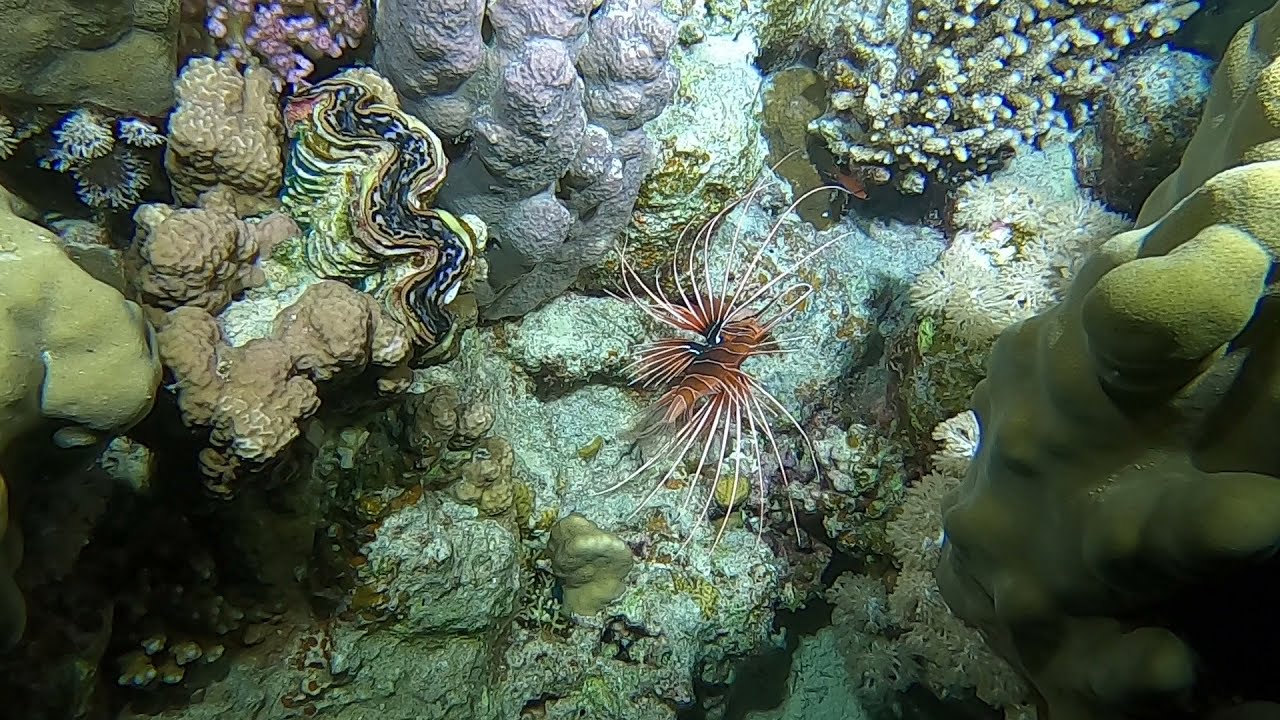The high-definition underwater photograph captures the ocean floor with a fascinating sea creature at the center. The creature exhibits a vibrant orange body, complemented by approximately 20 long, thin, pink legs extending from its front and back, adorned with intricate lines across its surface. It rests directly on a light green and light gray rock surface. Surrounding it, the seabed features a captivating array of colorful formations: to the left, a gray rock formation topped with purplish spheres and a water-like swirling formation. A smooth zigzagging blue line transitions into yellow, deep blue, and white hues in the center, adding more vibrancy. Above and to the right, there are light green algae-covered rock formations, and nearby, another section presents brown rocks. The upper right corner also reveals light green coral with small white circles at the tips, while the bottom corners of the image are shadowed, adding depth to the scene. The entire frame is rich with various shades of brown, turquoise, purple, and additional coral colors, highlighting the diverse underwater ecosystem.